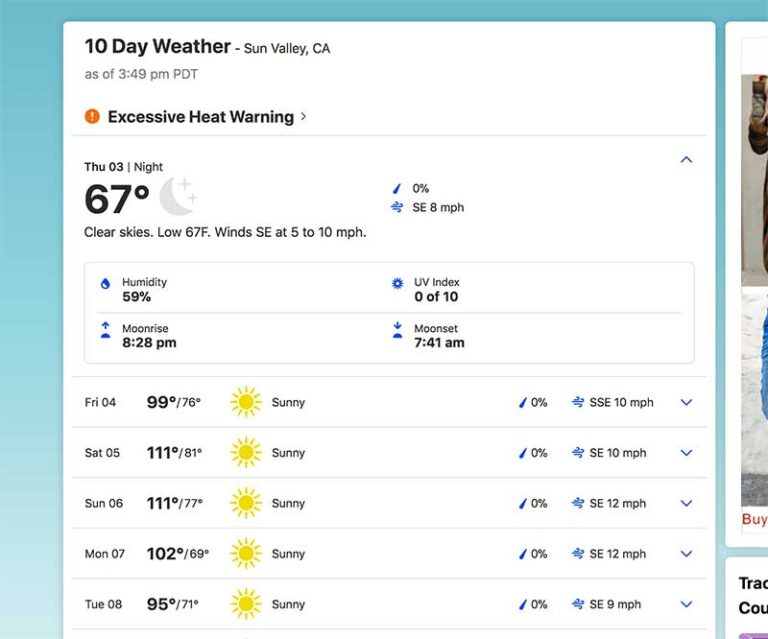The weather forecast display for Sun Valley, California, indicates a 10-day weather outlook. Current date and time are listed as 3:49 PM PDT. An orange exclamation mark denotes an "Excessive Heat Warning."

- **Thursday Night:** Low of 67°F, clear skies indicated by a gray, sparkly moon icon. Humidity: 0%, Wind: southeast at 8 mph.
- **Friday:** High of 99°F, low of 76°F, sunny, 0% chance of precipitation, wind from south-southeast at 10 mph. The UV index is 0-10. Moonrise at 8:20 PM, and moonset at 7:41 AM.
- **Saturday:** High of 111°F, low of 81°F, sunny, 0% chance of precipitation, wind from south-southeast at 10 mph.
- **Sunday:** High of 111°F, low of 77°F, sunny, 0% chance of precipitation, wind from south-southeast at 12 mph.
- **Monday:** High of 102°F, low of 69°F, sunny, 0% chance of precipitation, wind from south-southeast at 12 mph.
- **Tuesday:** High of 109°F, low of 71°F, sunny, 0% chance of precipitation, wind from south-southeast at 9 mph.

Other details include clear skies, currently a low of 67°F, with winds at 5-10 mph. The humidity, represented by a tear icon, is at 59%, and the UV index ranges from 0 to 10.